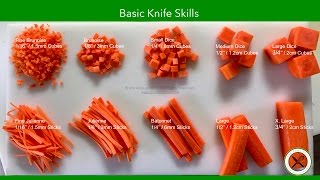In the image titled "Basic Knife Skills" displayed in vibrant Kelly green text, we observe various techniques of cutting carrots, which are bright orange and arranged meticulously. Starting from the top left, the carrots are finely shredded, transitioning to more coarsely grated pieces. To the right, there are neat, small cubes followed by larger, diced pieces, and finally, three uniform, square slices on the very top right. 

In the second row along the bottom, the leftmost section showcases thinly shaved carrot pieces, moving rightward to thicker carrot cuts. Continuing to the far right, the pieces become progressively chunkier, culminating in extra-large sections approximately three-fourths of an inch thick. Each style of cut is labeled in white text above the respective piles of carrots, and the entire presentation is framed with a thin Kelly green band at the bottom, featuring an X emblem on the bottom right corner.